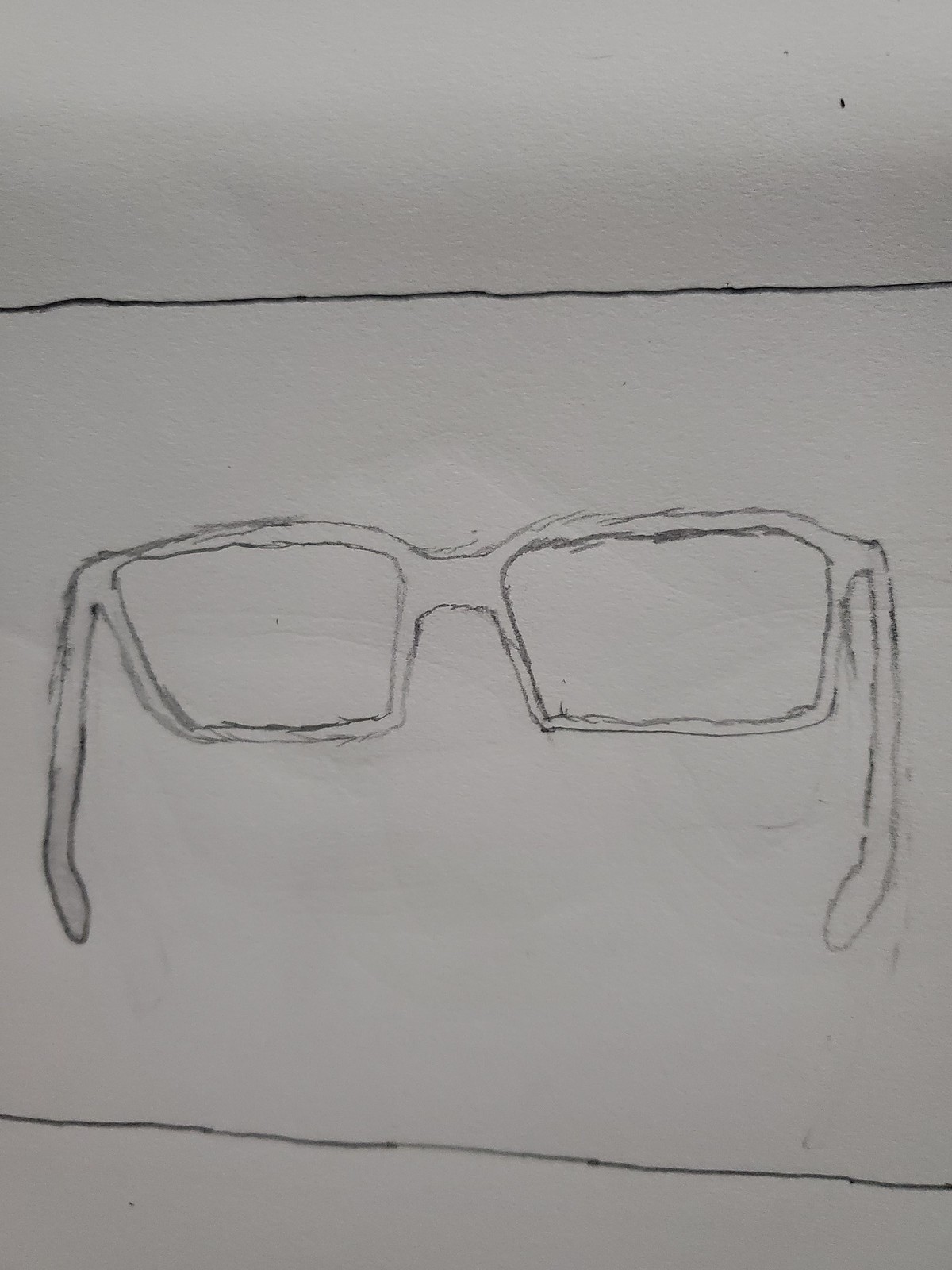The image depicts a photograph of a hand-drawn sketch on white paper. The drawing, executed in dark slate gray pencil, centers on a pair of glasses with flared rims and a distinct downward curve in the bridge and rims of the eyeglasses. The lenses appear somewhat rough and dynamic, adding a sense of motion to the otherwise static object. Across the page, there are two prominent horizontal lines—one situated about an inch above the glasses and another approximately an inch below them. These clean lines serve as borders framing the central depiction. There is no text on the image, which features only two colors: white and dark slate gray, creating a stark and minimalistic aesthetic.